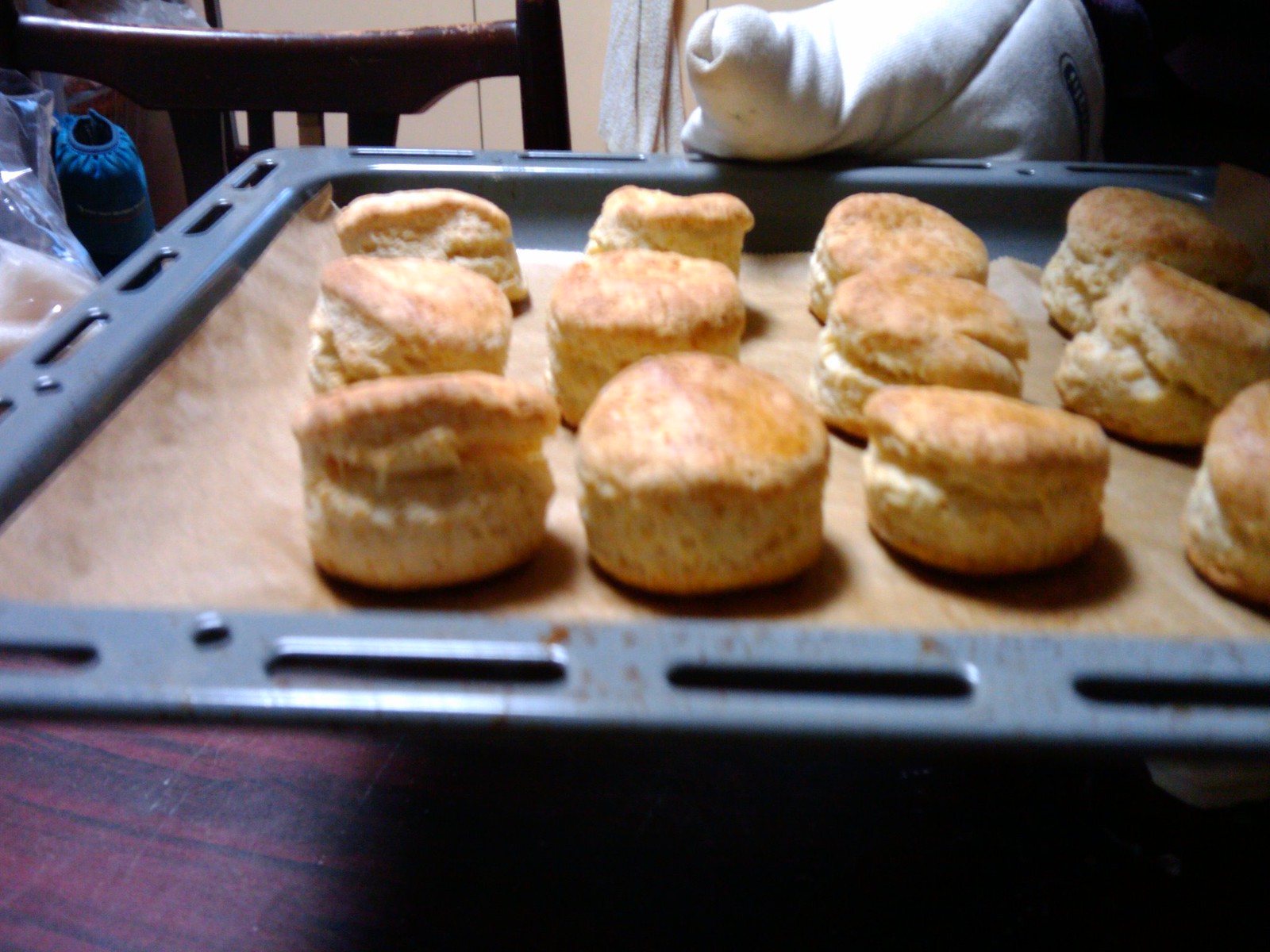This color photograph, taken in landscape orientation, captures a close-up of a baking tray holding 12 golden-brown, homemade tea biscuits, which have risen and split at the top. The biscuits rest on a sheet of parchment paper atop a gray metal baking tray, likely part of an oven. The image shows the hand of a person in a white oven mitt holding the tray at the top right corner, ready to place it on a wooden surface with a purple-blackish tint. Despite the slight blur and dim lighting, one can spot the back of a chair and a portion of a table in the background, suggesting the setting of a cozy kitchen or dining area. A hint of a yoga cover adds a touch of casual domesticity to the scene.